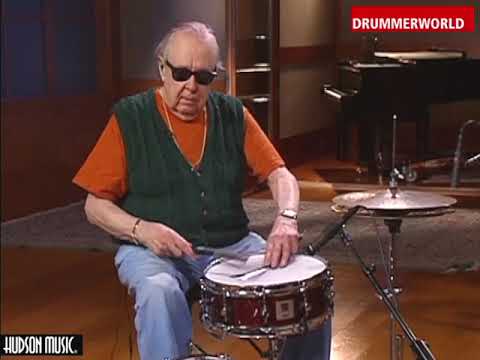The image is a detailed, full-color screenshot from a YouTube video, prominently featuring an older man, likely in his 60s, playing the drums. He is seated slightly off to the left and oriented towards the five o'clock position within a music studio setting. The man is dressed in a green vest over an orange short-sleeved t-shirt, blue jeans, black sunglasses, and a watch on his left wrist alongside a bracelet on his right. His thinning hair is noticeable, and he is holding drum brushes, suggesting he is performing jazz drumming techniques. He is positioned in front of a snare drum and a hi-hat cymbal, with a microphone leaning down to amplify the snare drum.

The background reveals various studio elements: a black baby grand piano with wooden paneling, a lighter hardwood floor partially covered by a large white throw rug, and some wood trim on the white walls. To the far left are visible doors and windows. The image is framed with a red banner in the upper right corner displaying "Drummer World" in white text, and a black banner in the lower left corner with the white text "Hudson Music," indicating the channels involved.